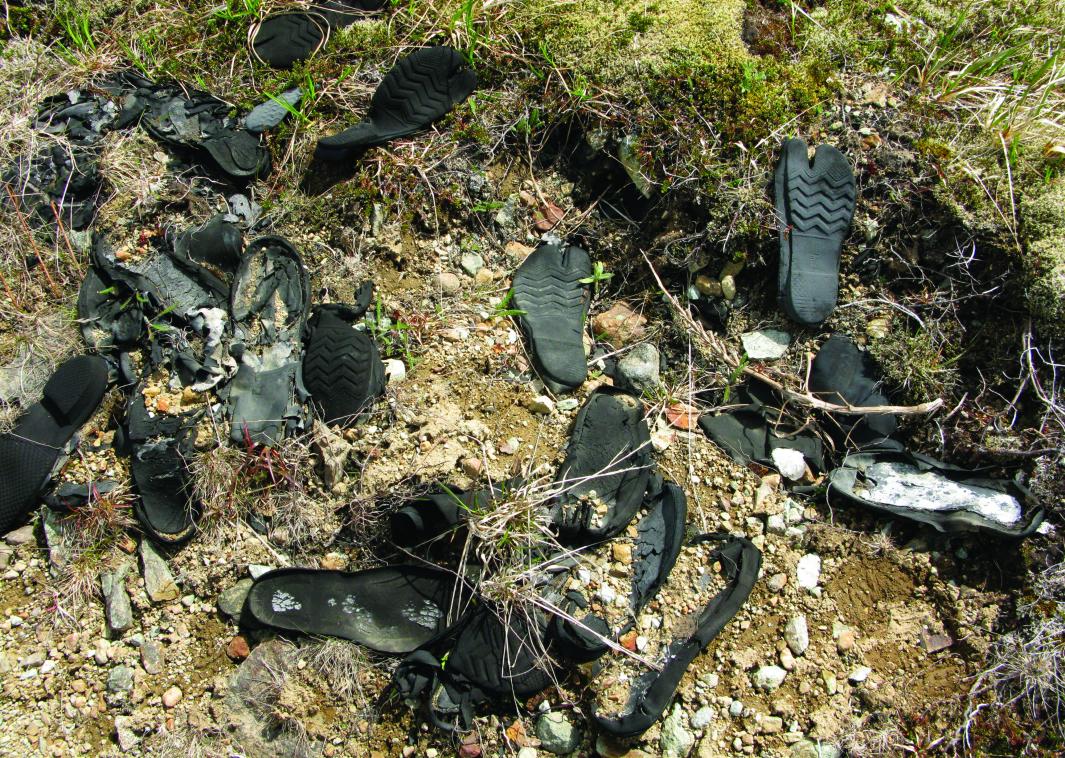The photograph captures an outdoor scene looking downwards at the ground, showcasing an embankment area reminiscent of a path leading to a riverbank. The setting is marked by a forest, a stretch of grass on a slight incline, and a patch of dirt and gravel. Scattered across this area are approximately 30 pieces of black rubber footwear, including soles from flip-flops and insoles from various types of shoes. The footwear appears to be in varying states of degradation and dirtiness, indicating they have been discarded for some time. Some of the rubber pieces seem partially buried, suggesting possible human intervention. The sizes of the footwear suggest they might have belonged to men. This assortment of discarded footwear suggests that someone has used this spot as an informal dumping ground.